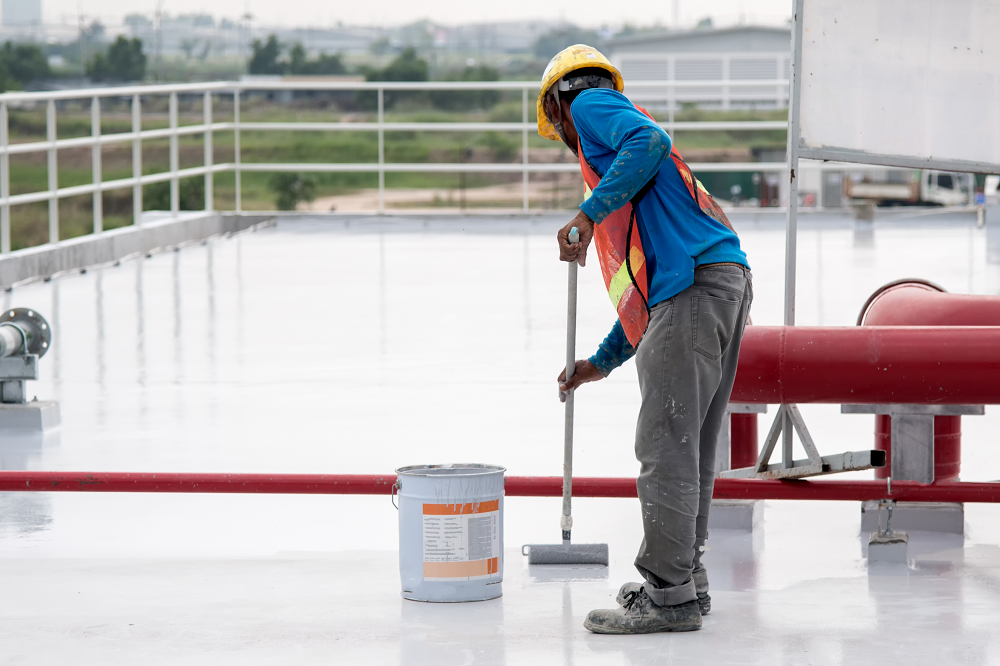The image shows a man working outdoors on what appears to be a rooftop on a cloudy day. He is painting the floor, which is shiny and gray, with a squeegee or a roller brush. The man is wearing a long blue sleeve shirt with an orange and yellow safety vest over it, black jeans stained with white paint, and paint-stained gray work shoes. He also has a yellow hard hat on and gloves for protection. In the background, there are buildings and a countryside view with green grass and trees. Surrounding the work area is a white fence and a railing. Notable items near him include a white bucket with an orange label, a red pole attached to a silver strap, and several red and gray horizontal bars and pipes. There's a gray pole with a sign, but the sign's details are obscured as it is shown from the back. A rock walkway is visible below the rooftop area.